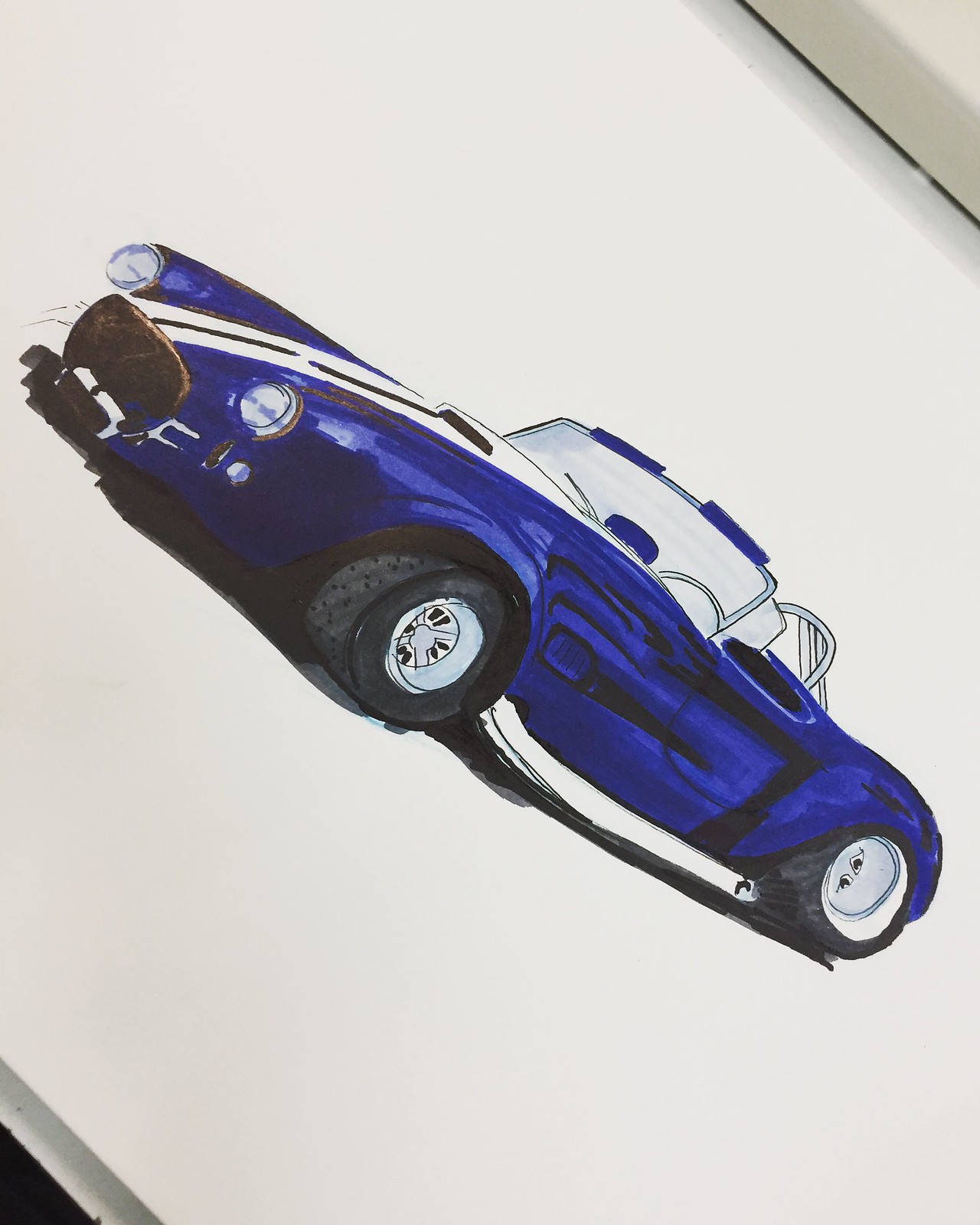The image showcases a detailed drawing of an antique blue sports convertible on a white sheet of paper, positioned on what appears to be a white desk or counter with a slightly off-white area at the top right suggesting part of the desk. The car is a low-slung, two-door coupe with a striking bright blue paint job and features two prominent white racing stripes running from the front bumper to the rear section. It has a distinctive chrome sidebar along its side, two chrome exhaust pipes, and black tires with silver wheels. Other noticeable features include a hood scoop, a windshield, a blue rearview mirror, and a white steering wheel. The car lacks a license plate and appears to be meticulously drawn to highlight its classic and sporty essence.